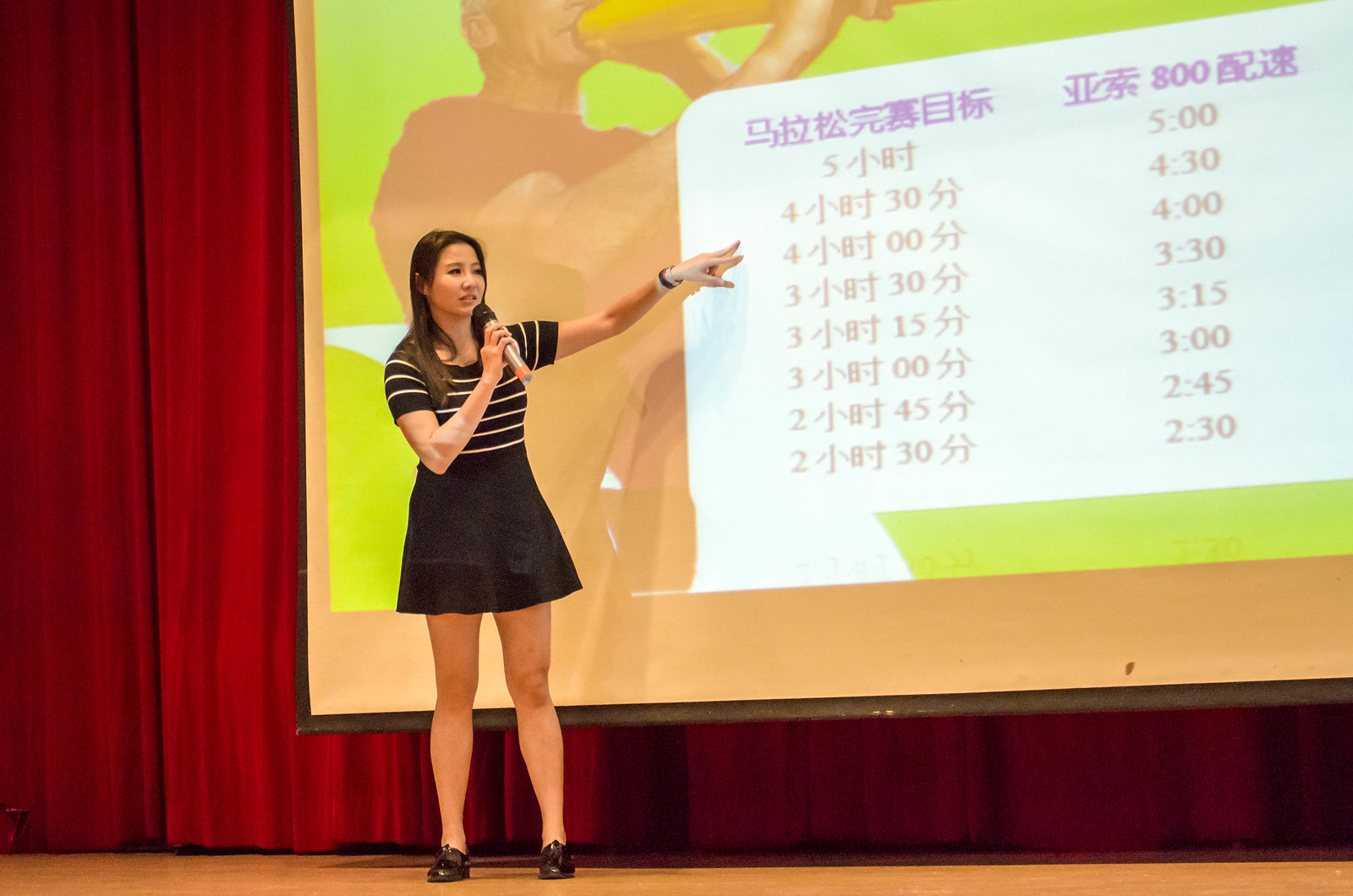In this image, an Asian woman is seen standing at the center of a stage, engaged in giving a presentation. She is holding a microphone in her right hand and pointing with her left at a large projector screen behind her. The projected image on the screen displays an older man, partially visible, with the lower half of his body shown holding something yellow, possibly a bullhorn. The screen also contains text in a different language, potentially Chinese or Korean, along with dates and times. The background of the projection is neon green. The woman, casting a slight shadow on the screen, has long black hair and is dressed in a black and white striped top paired with a black skirt and black flats. She also wears a watch on her left wrist. The stage itself has light brown, wooden flooring, and is set indoors with red curtains hanging behind the projector screen. The array of colors in the image includes light brown, tan, black, white, red, light green, yellow, gray, and blue, adding vibrancy to the indoor setting where the presentation is taking place.